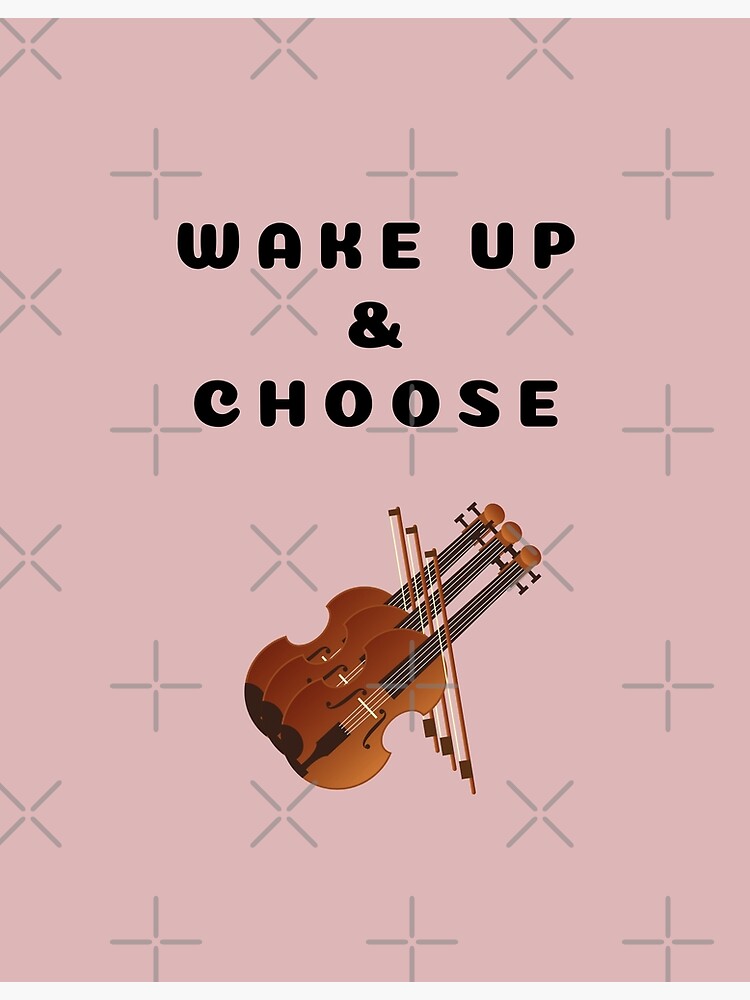The image is a vertically-oriented digital design with a dusky pink background. This background features an evenly spread pattern of grey shapes, including both X's and plus signs, reminiscent of diamond plate but more spaced out. Dominating the top third of the design, retro-style black bubble text reads "Wake up and choose." Just below this text are three overlapping violins rendered in a clip art or emoji style. The violins are positioned diagonally with their handles pointing towards the top right corner, and three bows are placed vertically on top of them in perfect alignment. The overall composition suggests a motivational poster.